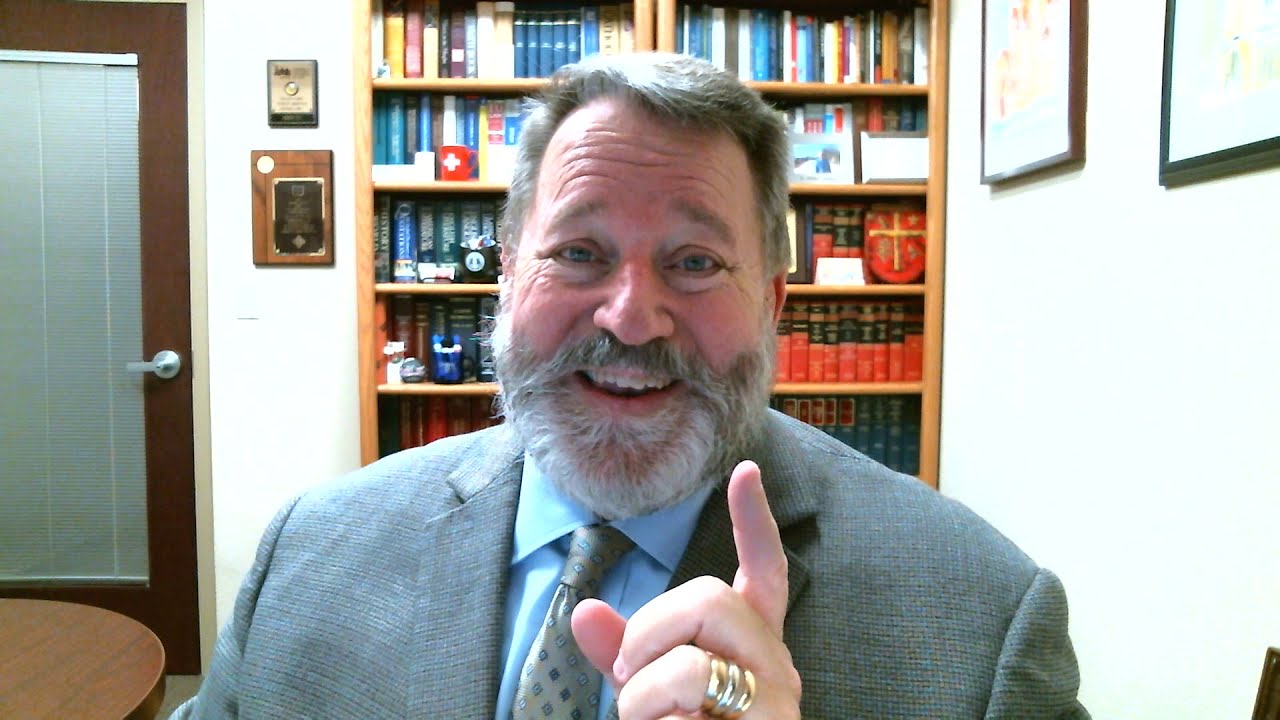This horizontal, rectangular image captures an older gentleman, probably in his late 50s, during what appears to be a Zoom meeting. Positioned centrally in the picture, he looks directly at the camera with a smile, displaying his teeth. He has salt-and-pepper colored hair, more white than gray, and a short, neatly-trimmed beard that is predominantly white with traces of brown. His hair is parted down the side, and he sports a mustache.

The man is dressed in a professional attire, including a gray suit jacket with a subtle square pattern, a blue collared long-sleeve button-down shirt, and a gray tie adorned with blue and darker gray diamond shapes. His left hand is raised in front of him, with his index finger pointed up as if he's making a point or answering a question. On his ring finger, he wears three gold bands.

Behind him, the room features white walls adorned with a couple of plaques and pictures on the right side. Two large brown bookcases, filled with books on every shelf, stand side-by-side directly behind him. To his left, part of a small round brown table is visible. A brown-framed door with blinds in its window and a silver handle is situated on the left side of the image. The overall setting suggests a scholarly or professional environment, adding to his authoritative yet approachable demeanor.